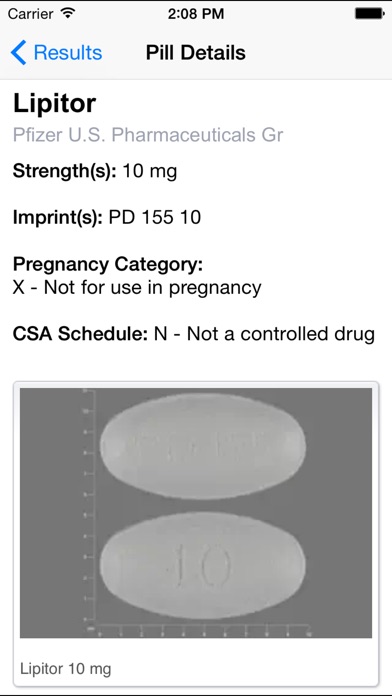The top of the screen features a black bar with a light gray header. On the top left, small dark gray or black font reads "Carrier." To the right of this, a black Wi-Fi symbol displays full signal strength. In the center, bold black text shows "2:08 PM." On the right side, an icon of a fully filled black battery indicates a full charge.

Below this header, on the left side, there is a large bold arrowhead pointing to the left. Next to it, non-bold blue text reads "Results." Centered below this, bold black text states "Pill Details," with each word capitalized. This section is housed within a white rectangular area, suggesting it could be part of an app or an email.

In the upper left corner of this white area, bold black text reads "Lipitor" (LIPITOR). Directly beneath it, in smaller light gray font, it says "Pfizer U.S. Pharmaceuticals GR." Below this, on the left, the term "Strength(s):" is written in bold black text, followed by "10 mg" in non-bold font. 

Further down, the label "Imprint(s):" in bold black text introduces "PD 155 10" in non-bold text. The following line reads "Pregnancy Category:" in bold black, with the information "X - Not for use in pregnancy" in non-bold font underneath.